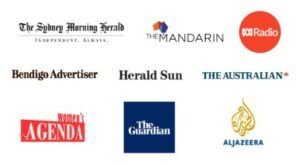This image is a promotional graphic for the Sydney Morning Herald, emphasizing a theme of independence. It includes an array of logos from various notable media outlets arranged neatly against a clean white background. The logos featured are as follows:

1. **The Mandarin Radio** - Displayed in white text within an orange circle.
2. **Bendigo Advertiser** - Icon not clearly described.
3. **Herald Sun** - Icon not clearly described.
4. **The Australian** - Written in aqua text with a small star next to it.
5. **The Agenda** - Embodied in white text with a red rectangle border.
6. **The Guardian** - Presented in white text within a blue square.
7. **Al Jazeera** - Showcased in blue text with intricate gold scriptwork and scroll designs inside the icon.

The image consists of a total of nine different logos, each representing a significant news outlet available in Sydney or across Australia. Each logo is distinctly designed, providing variety and a sense of global journalistic presence. The logos and text are relatively small and set against a simplistic white backdrop. The overall layout suggests it could be part of a web advertisement or possibly displayed on a mobile phone, although specific interface details are not visible.